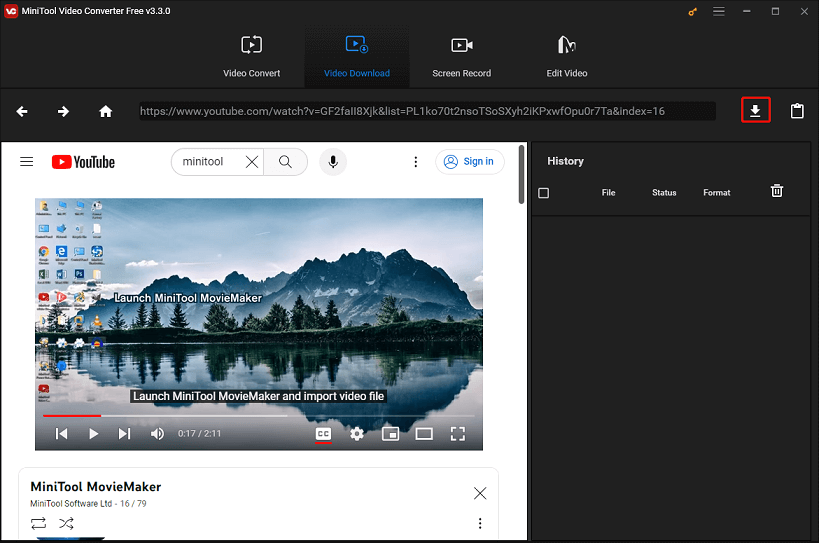Screenshot of a "MiniTool Video Converter" software interface on a computer screen. At the top-left corner, there's a red square icon with white text that appears to read "VC". Adjacent to it, the software name and version are displayed as "MiniTool Video Converter Free Version 3.3.0". Below this, a series of function boxes are visible, labeled "Video Convert", "Video Download", "Screen Record", and "Edit Video". 

The upper-right corner of the application window includes standard window control buttons for minimize, maximize, and close. Above the application, the web browser interface is visible with navigation controls, including back and forward arrows, a home button, and a URL bar displaying youtube.com followed by a long ID string. There's a prominent red "Download" button with a white download icon and a clipboard icon next to it.

Beneath the application window, the YouTube page reveals a search entry for "MiniTool". The user is not signed in, as indicated by the "Sign In" button. The video titled "MiniTool Movie Maker" by "MiniTool Software Limited" is playing, currently at 17 seconds out of a total duration of 2 minutes and 11 seconds. The scene shows a serene landscape with mountains, trees, and a lake, likely part of a demonstration within the tutorial video.

Further items on the screen include icons for applications like YouTube, Firefox, and others. To the right side of the screen, there are sections labeled "History", "File Status", and "Format".